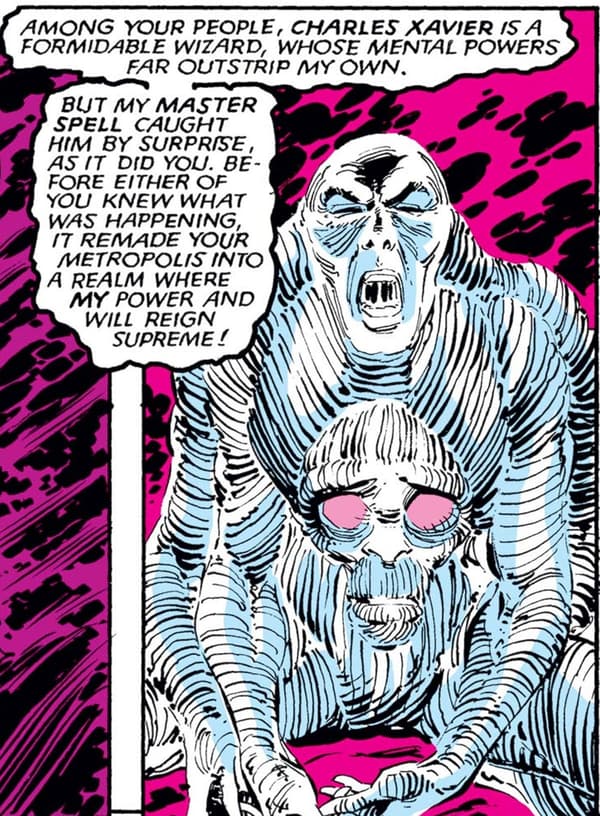The image depicts a color comic book illustration in portrait orientation. Dominating the right side is a black and white striped monstrous figure with multiple ripples along its neck, arms, and shoulders. Its face is contorted in a grimace, eyes squinted shut, and mouth wide open, revealing a wet, toothy snarl. Intriguingly, within its lower chest area, where one would expect a stomach, there appears to be another skull-like face with slightly apart lips and pink eye sockets, giving it a translucent, eerie effect. The backdrop is a vivid fuchsia with black irregular dot patterns reminiscent of an exaggerated cheetah print. At the top, a white speech bubble contains the text: "Among your people, Charles Xavier is a formidable wizard whose mental powers far outstrip my own. But my master spell caught him by surprise, as it did you. Before either of you knew what was happening, it remade your metropolis into a realm where my power and will reign supreme!" A white vertical strip beneath the speech bubble enhances the comic book feel of the illustration.